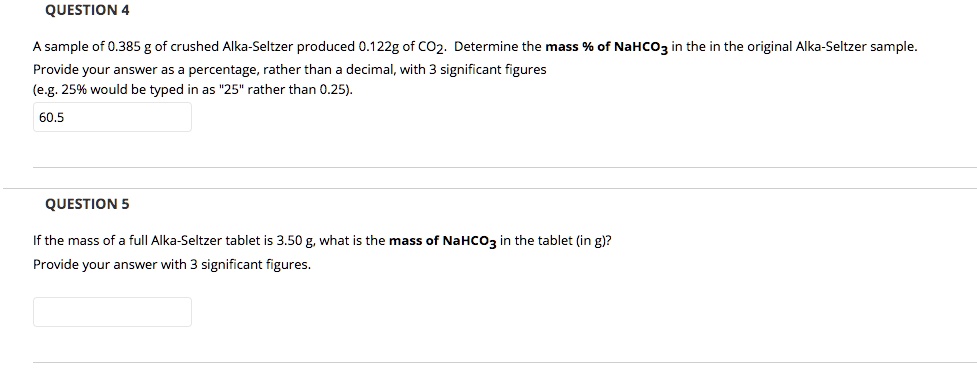Caption: 

On the left side of the image, black bolded text in all capital letters reads "QUESTION FOUR." Below this heading is regular black text stating: "A sample of 0.385 g of crushed Alka-Seltzer produced 0.11 g of CO₂. Determine the mass and % of NaHCO₃ in the original Alka-Seltzer sample. Provide your answer as a percentage rather than a decimal with three significant figures (e.g. 25% would be typed as '25' rather than 0.25)." 

Under this text, there is a horizontal rectangular box containing the number "60.5." Below the box are two horizontal light gray lines. 

Following this, another heading in bolded black text with "QUESTION" fully capitalized, and "Five" accompanying in the same font, is shown: "QUESTION FIVE." In regular black font, it asks: "If the mass of a full Alka-Seltzer tablet is 3.50g, what is the mass of NaHCO₃ in the tablet (g)? Provide your answer with three significant figures."

There is another horizontal rectangular box below this question, which is currently empty. At the bottom of the page, there is a horizontal light gray line.